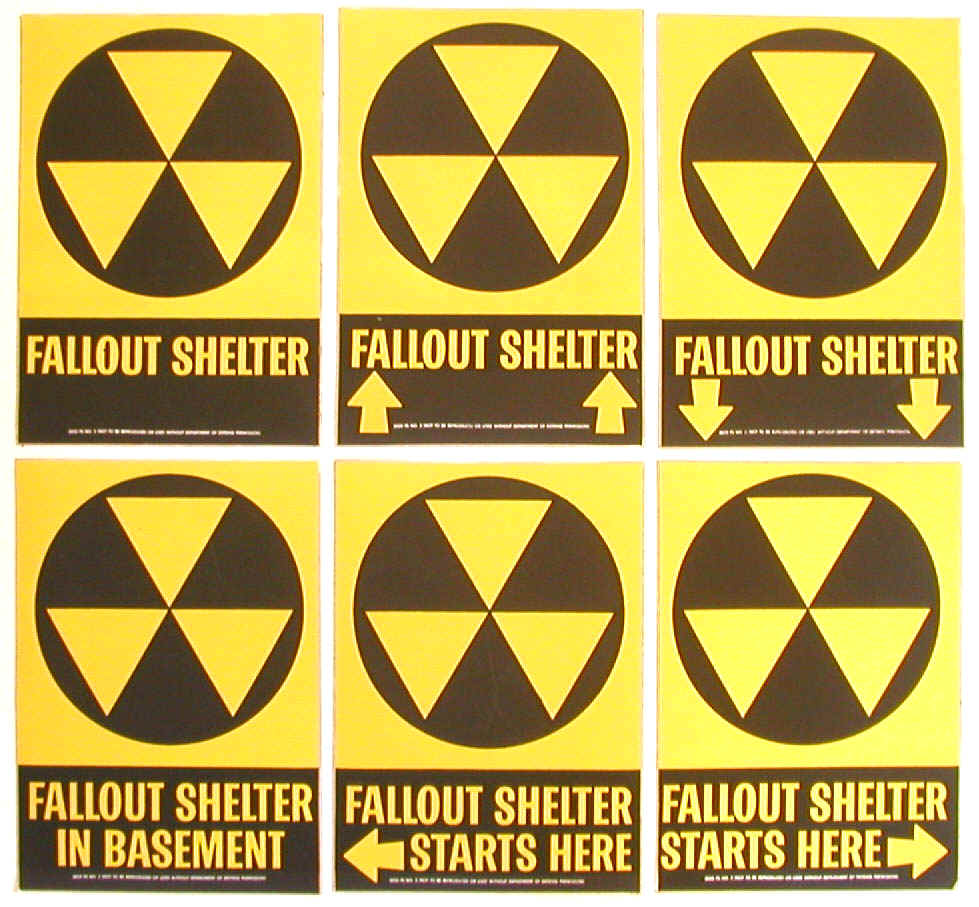The image contains six different Fallout Shelter posters, each featuring a yellow background with a prominent black circle at the top, inside of which are three upside-down yellow triangles. The lower half of each poster has a black background with yellow text. The first poster simply states "Fallout Shelter." The second poster also says "Fallout Shelter" but includes two yellow arrows pointing upwards. The third poster is similar but with two yellow arrows pointing downwards. The fourth poster has the text "Fallout Shelter" with an additional line stating "In Basement." The fifth poster has "Fallout Shelter" and the text "Starts Here" accompanied by a yellow arrow pointing left. Finally, the sixth poster mirrors the fifth but with the arrow pointing to the right. Each poster serves as a directional or informational guide for Fallout Shelter locations, with subtle differences in the designs and instructions to cater to various scenarios.